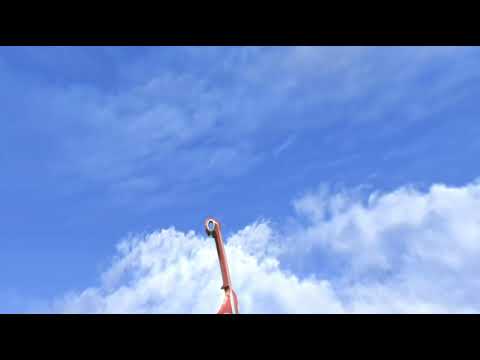The photograph captures an upward-looking perspective at the top of a white flagpole, which is topped with a small tan circle, approximately a couple of inches in diameter. At the bottom of the pole, a small part of a red flag tip is visible against the sky. The picture is framed by a deep blue sky adorned with thin, transparent clouds at the top gradually transitioning to thicker, darker gray clouds in the bottom right corner. The image appears to include black bands at the top and bottom, adding a framed look to it. Despite some confusion in the descriptions, it is clear that the photograph was taken during the daytime and showcases a primarily blue sky with varying cloud densities, highlighting the flagpole's structure and emphasizing the contrast between the man-made pole and the natural sky backdrop.